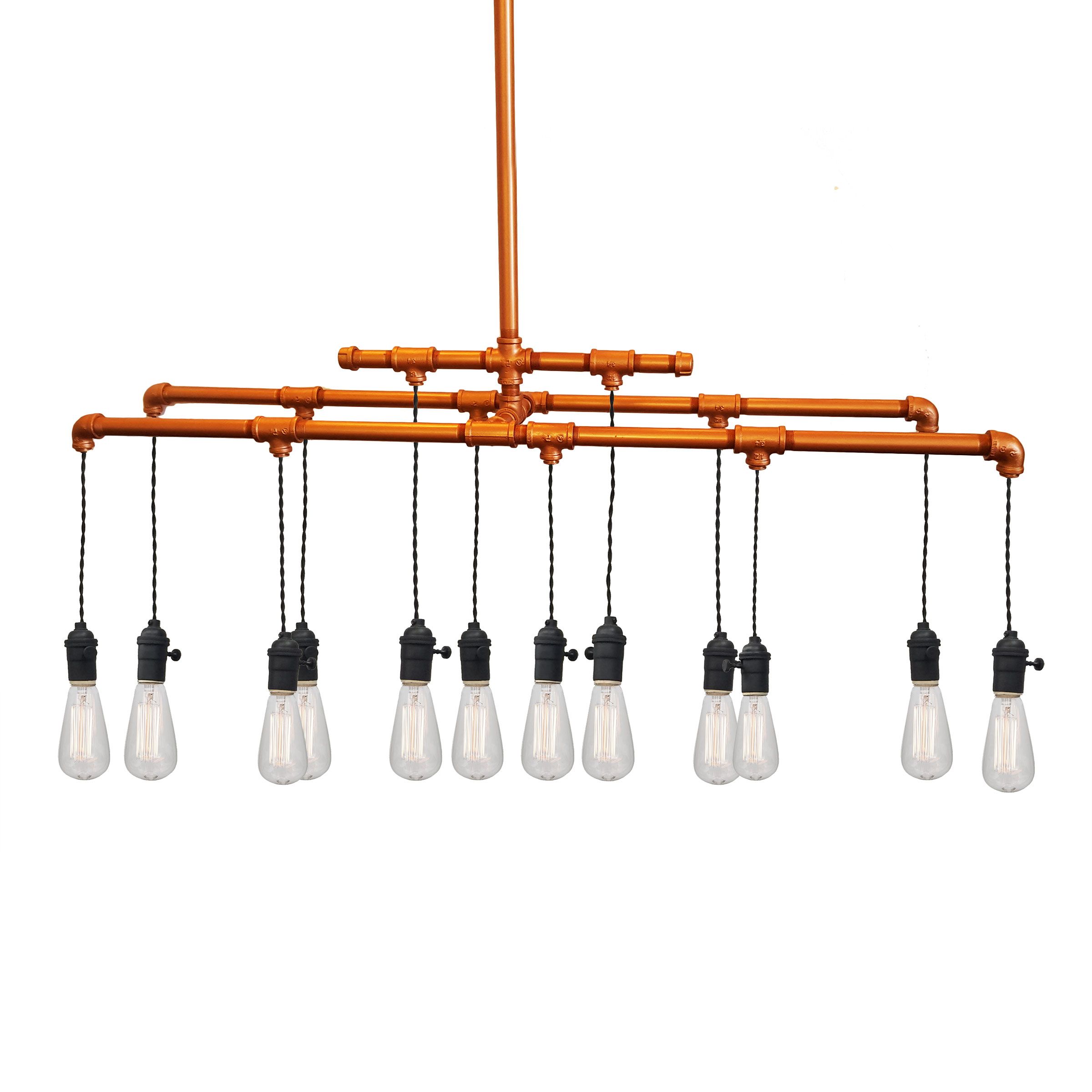This image appears to be a detailed drawing of a unique light fixture composed of bright orange metal pipes and vintage-style light bulbs. The fixture features three rows of pipes: two main rows and one smaller upper row holding two light bulbs each. The arrangement includes a total of twelve bulbs that hang down from the pipes, with the majority concentrated in the middle row in a pattern of four bulbs flanked by two bulbs on either side, for a two, two, four, two, two configuration. The entire setup is viewable against a pure white background, providing stark contrast to the fixture. The bulbs are either modern LEDs designed to look vintage or possibly authentic vintage models, and some of them even include an on-off switch at their base. The pipes converge into a central pole, presumably for wiring purposes, giving the drawing a symmetrical and cohesive appearance.